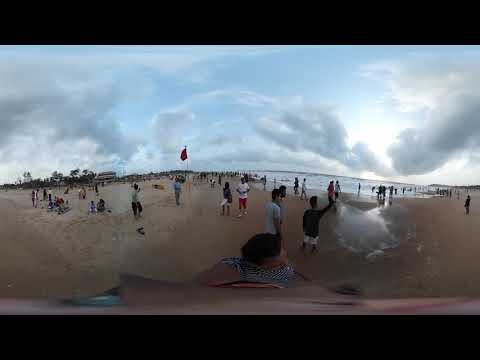This image captures a vibrant, partly sunny beach scene bustling with activity under a sky dotted with various clouds. The beach stretches across the horizon, meeting a somewhat wavy ocean in the distance. Numerous people, easily exceeding a hundred, are scattered across the sandy shore. They are engaged in various activities, such as walking near the water, sitting on blankets, or lounging on chairs, dressed in casual summer attire. 

In the center left of the image, a prominent red flag stands, possibly indicating a lifeguard station or storm warning. Near the foreground on the right side, a man in white shorts and a dark sweatshirt is pointing towards the sky, seemingly explaining the cloud formations to a young companion. To the left, another person sits close to the camera, their back turned, with black hair visible. Further along, a person in a black t-shirt and white shorts raises their hand, possibly holding a transparent and white balloon or bubble, adding to the playful atmosphere.

In the extreme distance on the left, a few buildings and palm trees can be seen, anchoring the scene as they blend into the cloudy yet bright daytime sky. The photograph appears slightly distorted, likely taken with a wide-angle lens, emphasizing the expansive and dynamic nature of this beachside gathering.